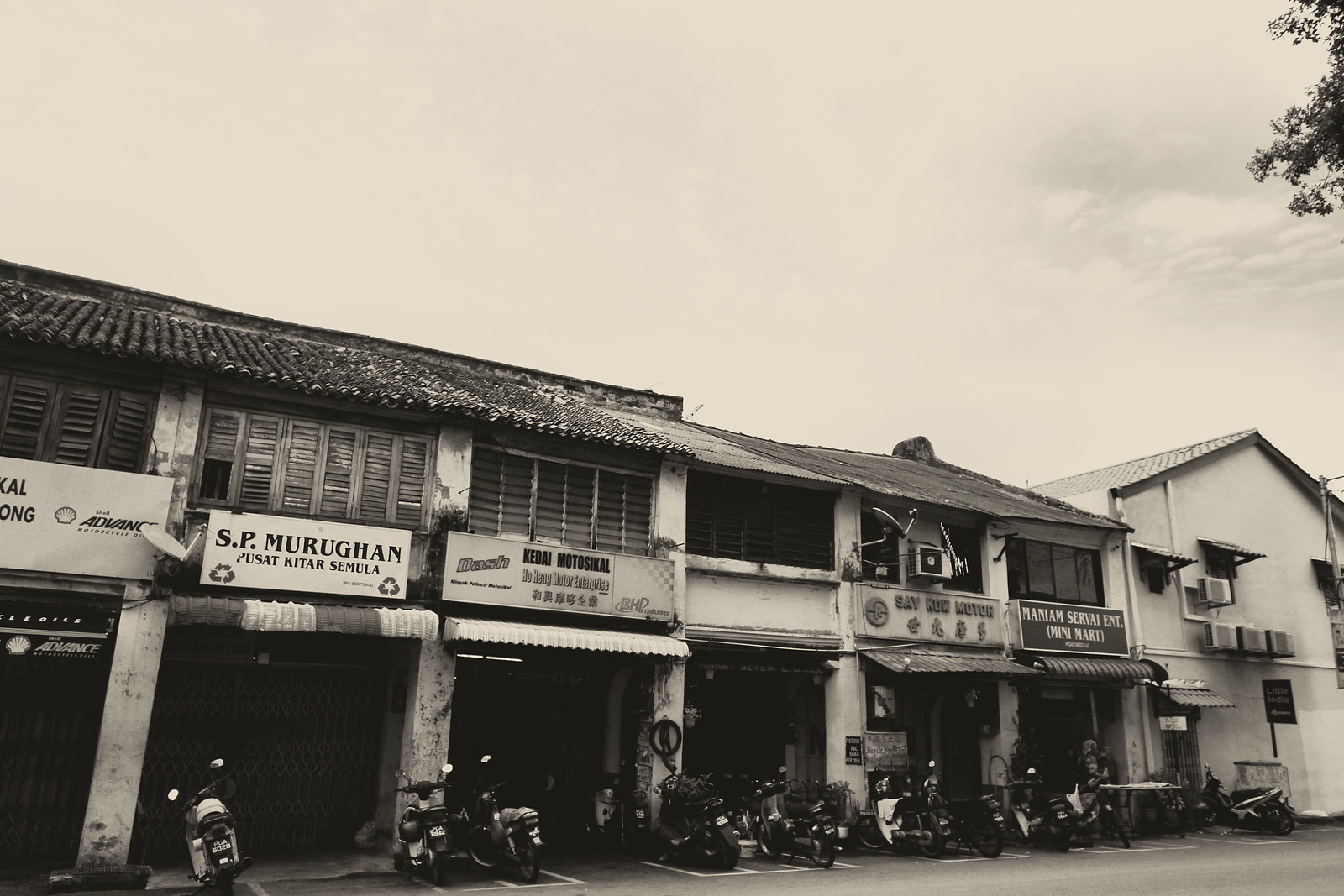The black-and-white photograph captures a nostalgic scene of a street lined with six connected storefronts forming a single, long, two-story building. This building, characterized by its varying roof styles—a rounded tile roof on one section and a straight one on another—extends from the left side of the image towards the right. The leftmost storefront is cut off at the edge of the photograph, displaying only half of it, while the far right showcases a separate white-walled building with four visible air conditioning units protruding from its side.

Each storefront features signage in a non-English language, though legible details are scant, apart from a partial reading of "S.P. Mergen." These signs indicate the presence of diverse businesses, though specifics remain unknown. Parked in front of the six storefronts are numerous motorcycles—at least ten—neatly arranged in rows, suggesting marked parking spaces possibly intended for two-wheeled vehicles.

In the bottom foreground, the image reveals a marked street area, again hinting at designated parking. The sky above is predominantly overcast with clouds, but a hint of tree branches adorned with leaves intrudes from the top right corner, adding depth to the scene. A single individual can be seen standing near the first storefront on the far right, enhancing the image's historical and communal atmosphere.